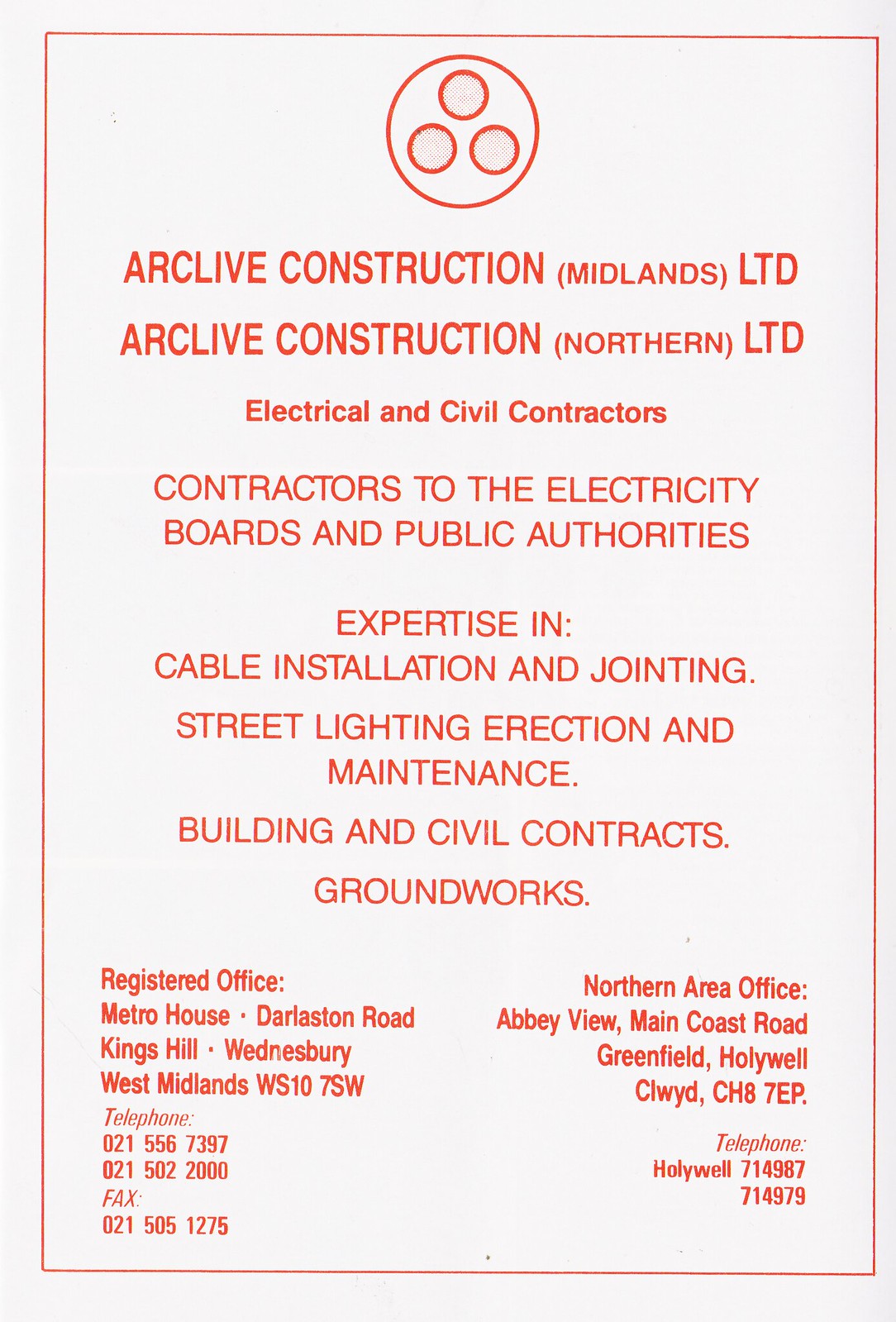The image is a tall, rectangular flyer with a light gray background and an orange-bordered inner rectangle. At the top, there's an orange-outlined round button with three holes. The flyer prominently reads in orange font: "Arklive Construction, Midlands LTD" and "Arklive Construction, Northern LTD." It details the company's services including electrical and civil contracting, working with electricity boards and public authorities, cable installation and jointing, street lighting erection and maintenance, building and civil contracts, and groundworks. At the bottom, it lists the contact information: the registered office at Metro House, Darliston Road, Kings Hill Wednesbury, West Midlands, WS10 7SW, Telephone: 021-556-7397, 021-502-2000, Fax: 021-505-1275, and the Northern Area Office at Abbey View, Main Coast Road, Greenfield-Holywell, Clywood CH870P.